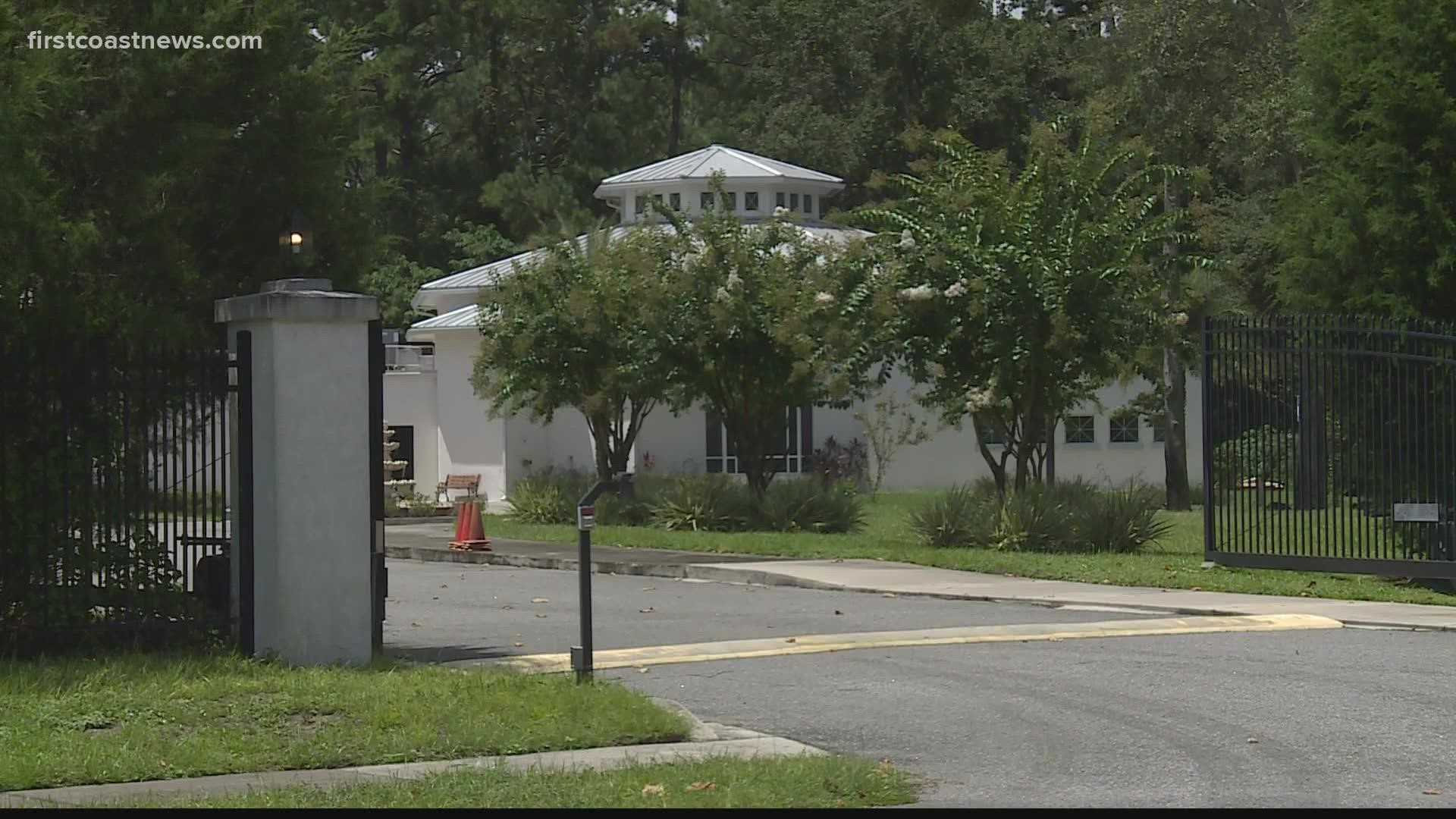This horizontally aligned rectangular photograph captures a picturesque white stucco house, possibly located in a coastal and affluent neighborhood, as indicated by the "firstcoastnews.com" watermark in the upper left corner. The house, which might be one or two stories high, features a distinctive hexagonal observatory-style structure with a hipped roof and windows on all sides at the top. 

Surrounding the residence are numerous tall, verdant trees, many of which appear to be evergreens, implying a spring or summer setting. The house is nestled within a well-maintained green grassy yard, prominently featuring three distinct trees in the foreground.

The property is enclosed by a tall, 10-12 feet high, black wrought iron fence with a large, open double gate. Adjacent to the gate are grey columns topped with lamplights, which are lit despite the bright daytime setting. The road leading to the house is grey with visible tire marks and a yellow-striped speed bump.

In the lower left corner, there is a sidewalk bordered by grass, where a few red safety cones suggest ongoing work. In the background, a bench and additional trees are visible, further enhancing the tranquil, leafy ambiance of the scene.